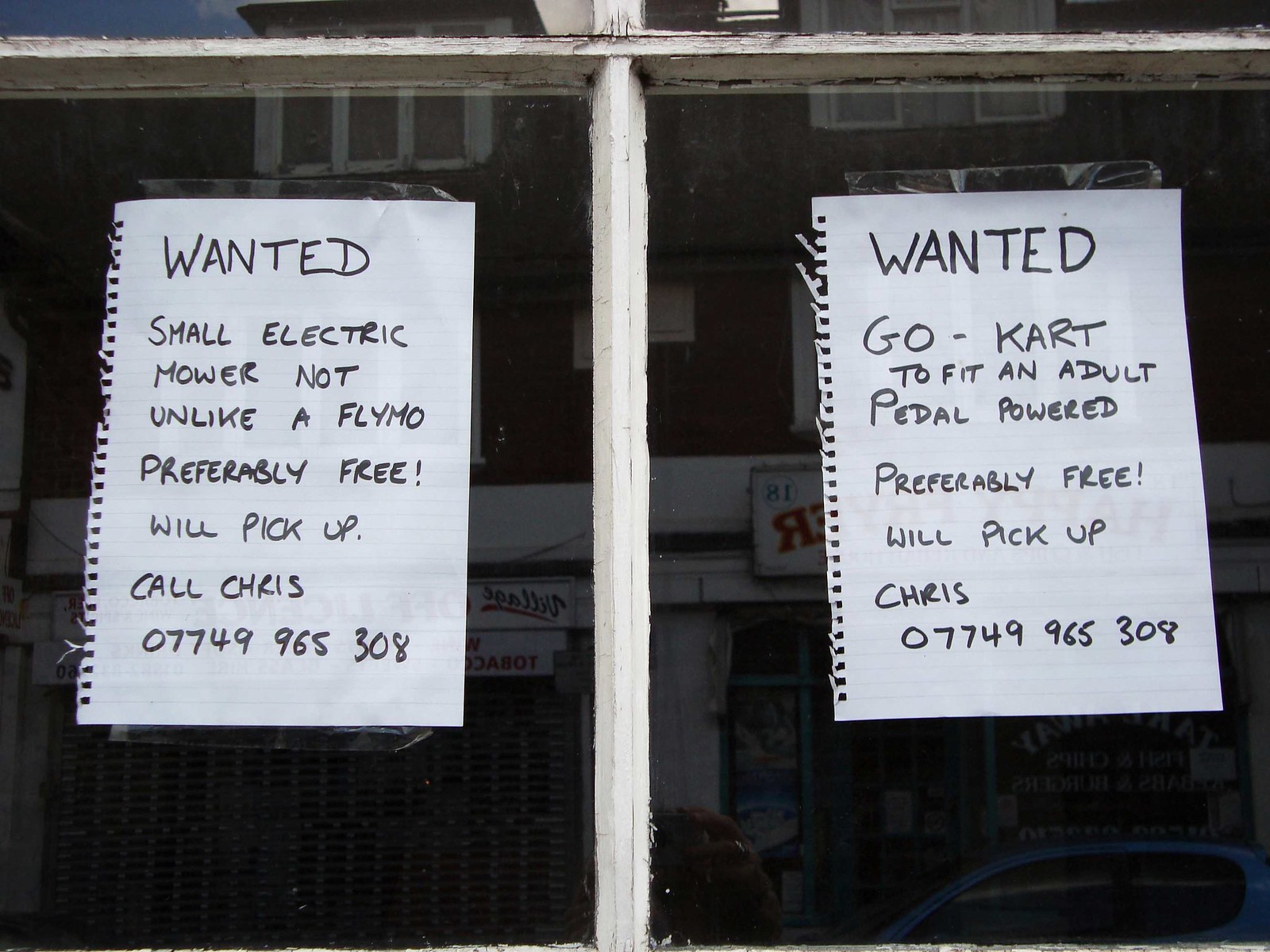This image captures a pair of handwritten notices taped to the panes of a weathered, white-painted wooden window frame, which seems somewhat rotted from exposure. Both notes are raggedly torn from spiral notebooks and affixed with clear cellophane tape. The left page reads: "Wanted, small electric mower not unlike a Flymo, preferably free. Will pick up. Call Chris, 07749-965-308." The right page mirrors the style, stating: "Wanted, go-kart to fit an adult, pedal powered, preferably free. Will pick up. Call Chris, 07749-965-308." In the background, reflected in the window, faint outlines of surrounding buildings and street signs are visible, adding an urban context to the scene.